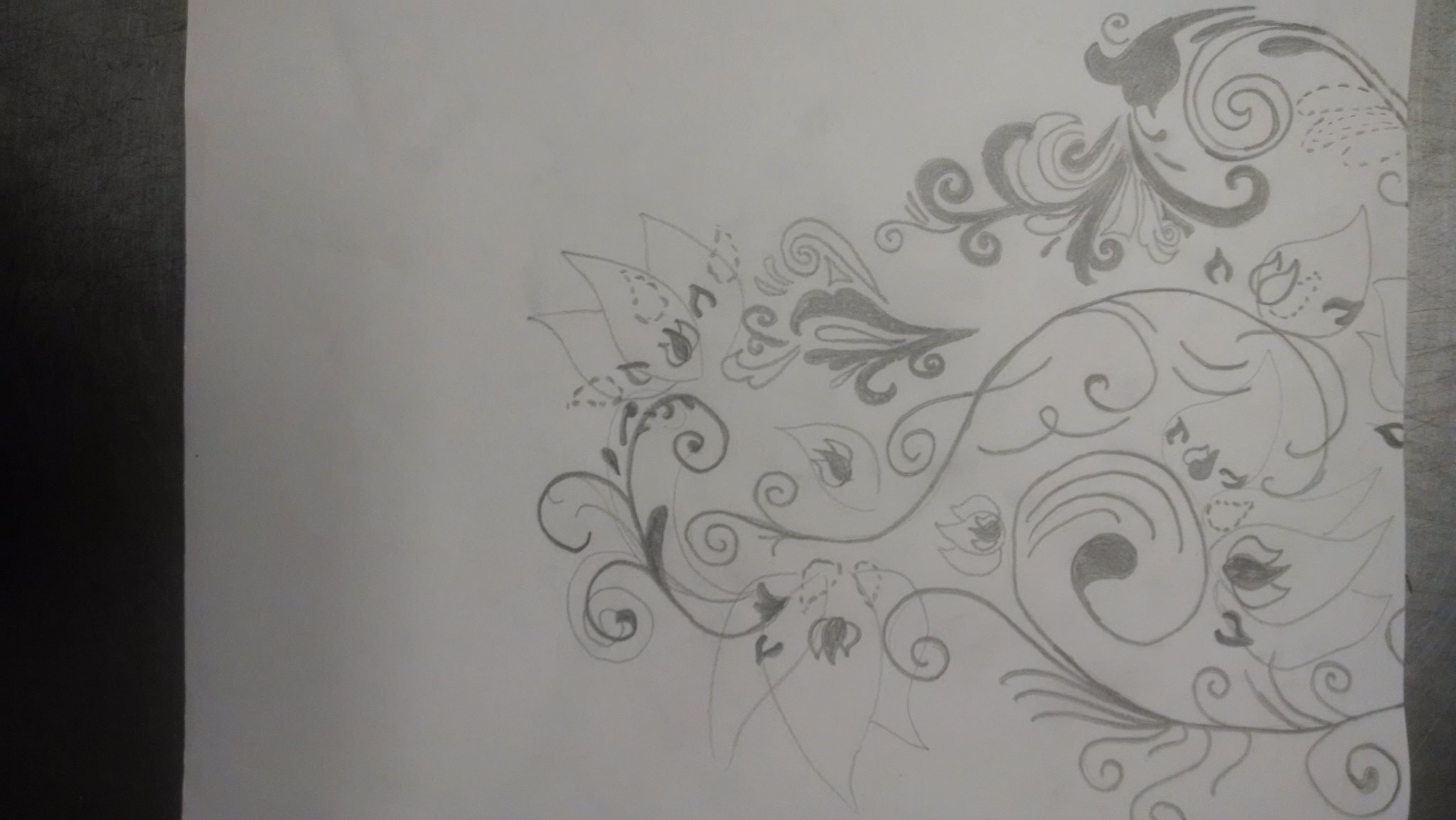This image showcases a hand-drawn artwork rendered in pencil, presenting a detailed, black-and-white composition. The drawing features intricate, vine-like tendrils that meander gracefully across the page, culminating in delicate flowers at the ends of the vines. The entire drawing occupies roughly three-fifths of the white paper canvas. Upon closer inspection, it seems that the piece is not entirely finished; a central flower appears incomplete, lacking full detail and shading. The overall aesthetics of the piece are characterized by its intricate, twisting vines interspersed with unfinished floral elements.